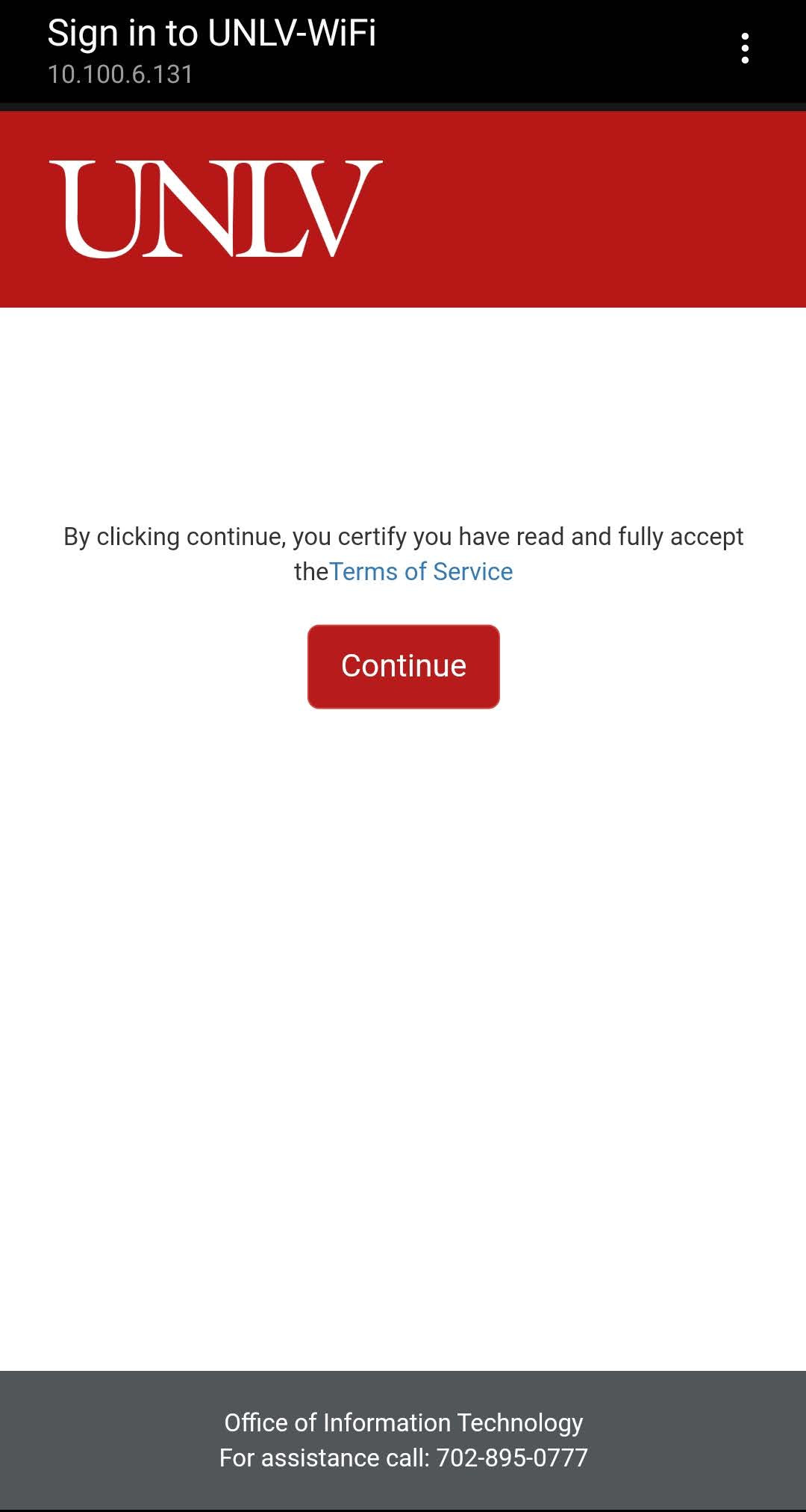The image is a screenshot taken on a phone, displaying an interface for connecting to the University of Nevada, Las Vegas (UNLV) Wi-Fi network. At the top of the screenshot, a narrow black bar (occupying about 5% of the image) contains white text that reads, "Sign into UNLV Wi-Fi," followed by an IP address: "10.100.6.131." Below this, a larger red bar prominently features the university's acronym, "UNLV," in uppercase, large white text.

The central portion of the screenshot is dominated by a large white section, within which, approximately in the middle, there is smaller gray text stating, "By clicking continue, you certify you have read and fully accept the terms of service." The phrase "terms of service" is highlighted in blue, indicating it is a clickable link leading to further details. Directly below this text, there is a conspicuous red button with "Continue" in white text, inviting users to proceed.

Finally, the bottom of the image is capped by a medium gray bar with white text, which reads, "Office of Information Technology for assistance call 702-895-0777," providing users with a contact number for technical support.